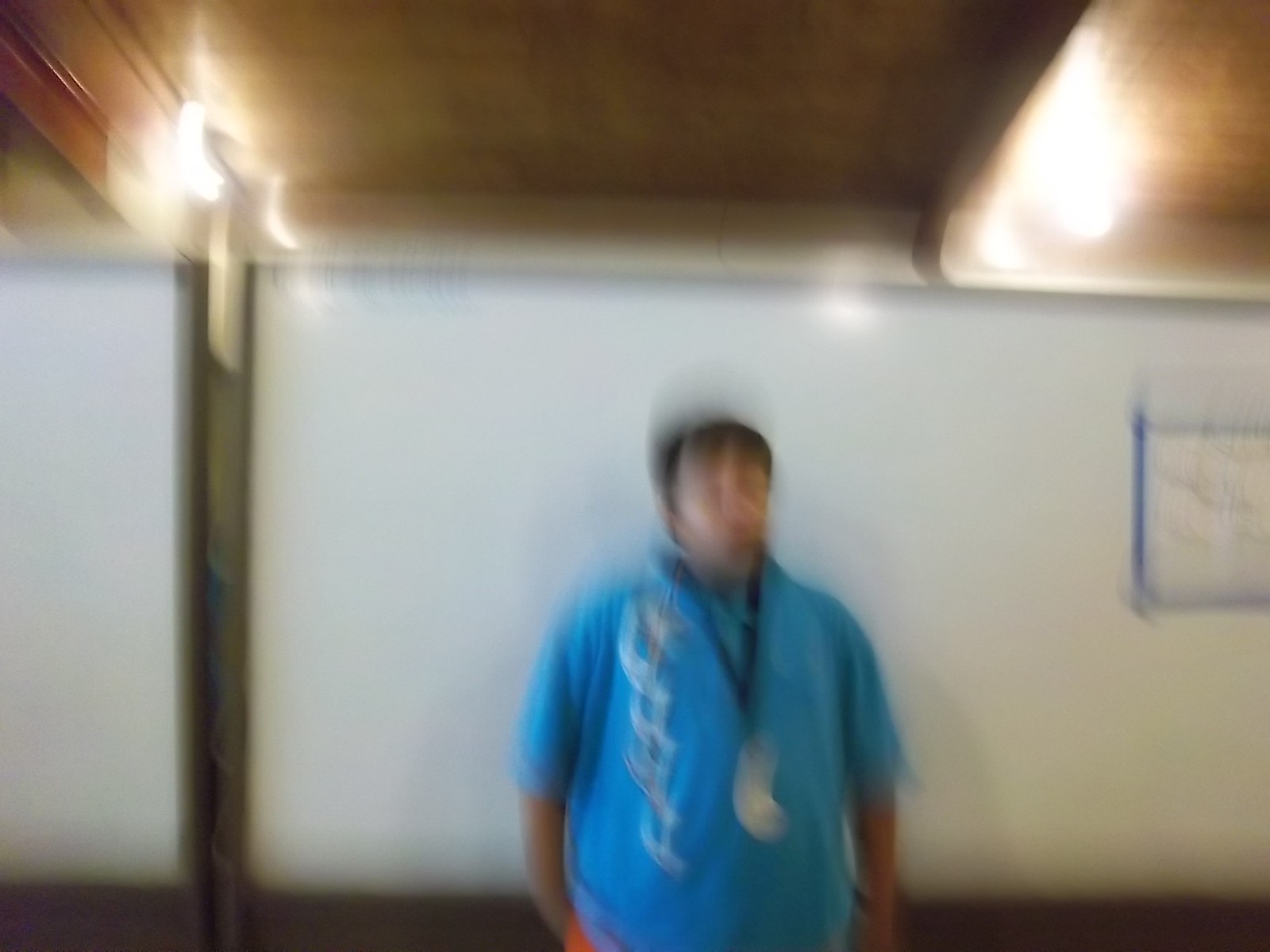In this blurry photograph taken inside what appears to be a basement or a room with wooden ceiling beams, a man with short dark hair stands in front of a whiteboard. The whiteboard has something taped to it with blue painter's tape. The man, possibly a teenager, has a slightly pale, perhaps light-skinned Hispanic complexion and is wearing a blue collared shirt that features a design detail on his right shoulder. He sports a large, metal lanyard-style necklace around his neck. His stance shows one hand in his pocket while the other rests by his side. He stands evenly spaced between two ceiling lights and positions himself just to the right of the camera, not looking directly at it. To the right of the man is a blue-bordered box or picture on the wall, with a small brown pole or divider nearby. The setting, combined with the man's casual attire and partially obscured face, gives an overall impression of an informal indoor environment.